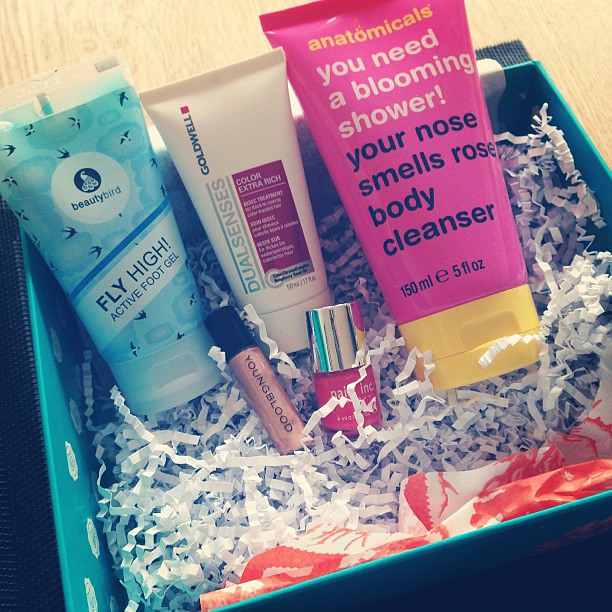The image features a teal beauty subscription box filled with white confetti and orange and white tissue paper, resting on a pale wooden table. Inside the box are multiple beauty and personal care products: a large hot pink bottle with a yellow cap labeled "Anatomicals - You Need A Blooming Shower, Your Nose Smells Rose Body Cleanser"; a blue tube labeled "Fly High Active Foot Gel" with the Beauty Bird logo; a white bottle with a purple bar containing ingredient details and labeled "Goldwell - DualSenses, Color Extra Rich"; a hot pink nail polish with white text and a silver cap; and a slim pale pink tube with a black cap labeled "Youngblood."